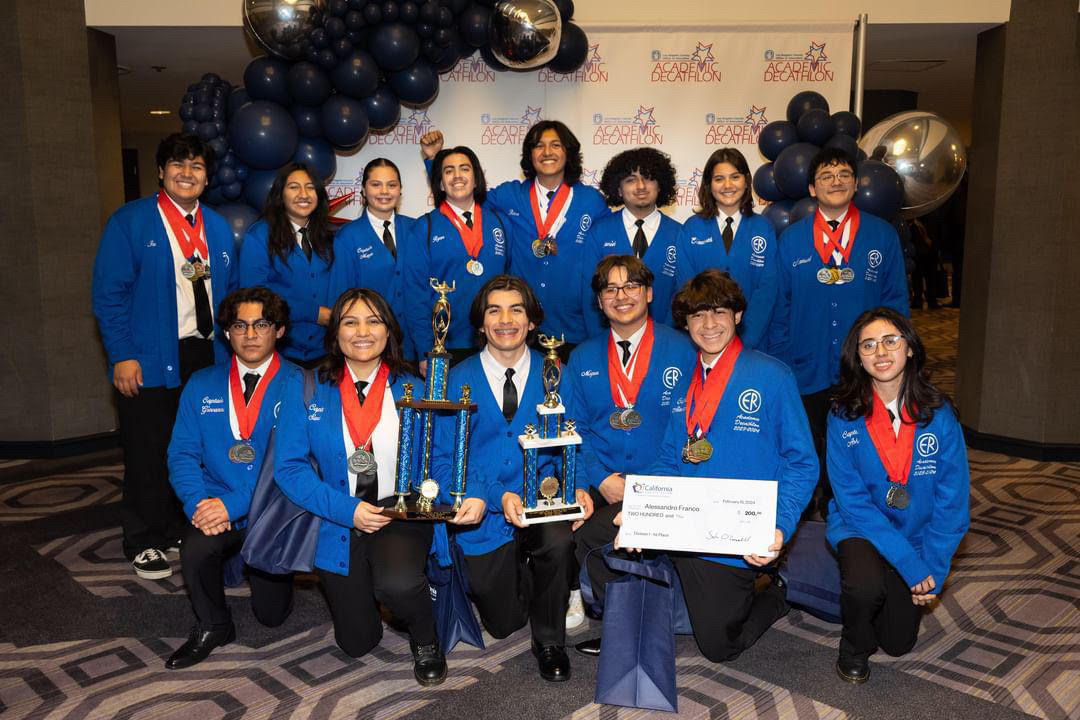This is a horizontally oriented photograph of a jubilant student team celebrating a recent victory in an academic decathlon. The image captures about 15 boys and girls, all clad in royal blue jackets emblazoned with the letters "ER" enclosed in a round circle. Beneath their jackets, they don white shirts, black ties, and black slacks, with footwear varying between black and white sneakers and plain black shoes. Each student proudly wears a red lanyard with medals hanging from the end, signifying their achievements.

The arrangement includes two rows: a group of students kneeling in the front and another standing behind them. Centered in the front row, a girl with a beaming grin holds a large trophy, while next to her, a boy brandishes a slightly smaller trophy. To their right, another boy kneels, prominently displaying a large paper check, suggesting a monetary award. The scene is set on a grayish carpet with subtle patterns, inside a building.

Behind the students, a backdrop adorned with the words "Academic Decathlon" hints at the nature of their accomplishment. Complementing the celebratory atmosphere, black balloons dangle to the left of the backdrop, and a doorway is visible, leading to another room where more people can be seen. Adding to the festive mood, one student in the background raises his fist in a victorious gesture.